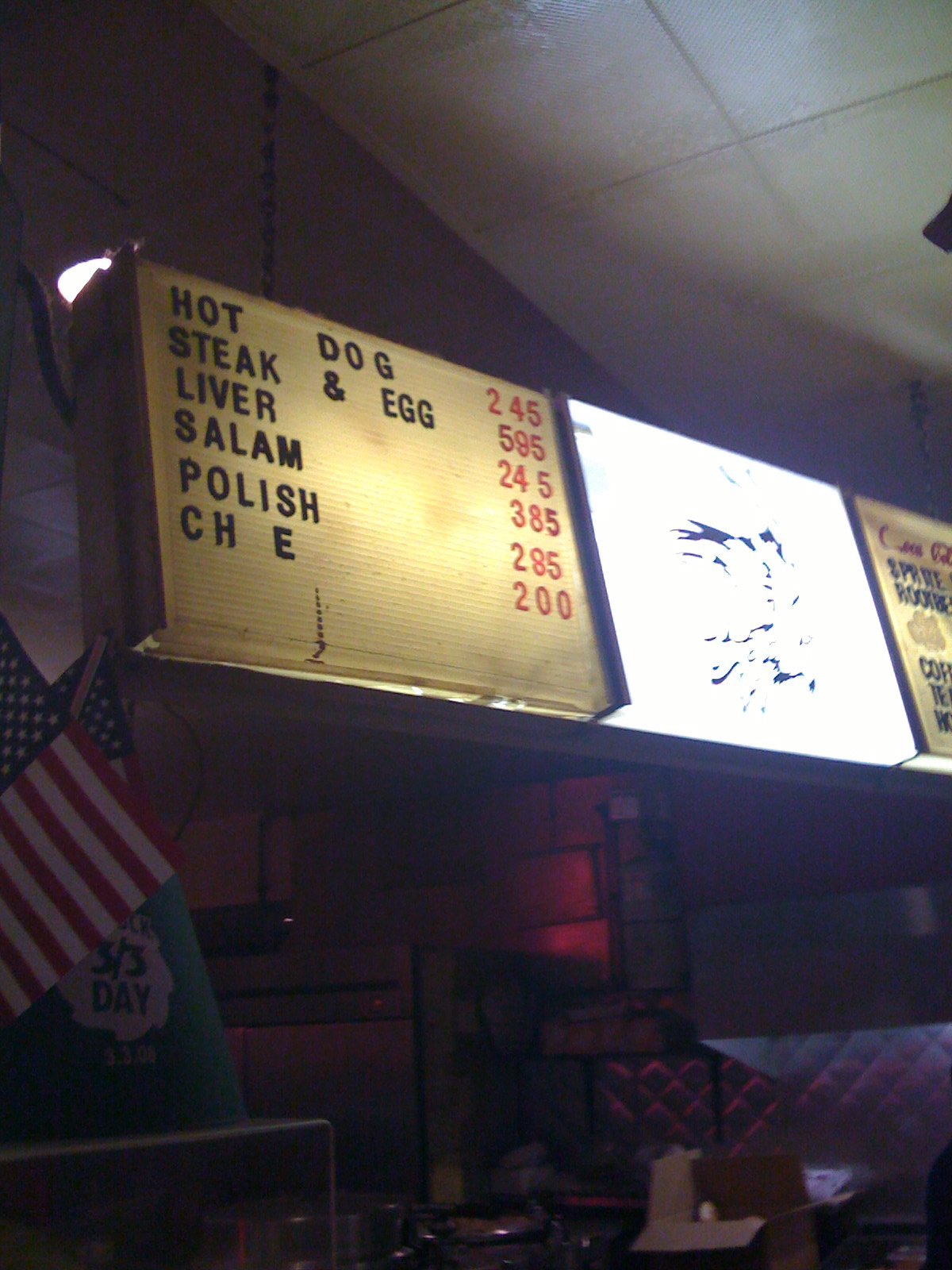In this vintage scene, a well-worn, illuminated plastic menu sign reminiscent of the 1960s through the early 2000s is prominently displayed, characteristic of delis and walk-in restaurants from that era. The sign is purely mechanical, allowing for prices and items to be changed by manually inserting letters and numbers into the grooves, devoid of any digital or LED technology. This classic sign lists menu items like hot dogs, steak and eggs, liver, salami, Polish sausage, and an item partially obscured as "CH  E," with prices ranging from $2.45 to $5.95.

Below the sign, a stainless steel flat top grill surrounded by a similarly stainless steel frame suggests an active food preparation area, typical of a small, independently-owned American deli or fast-food establishment. An American flag adorns the wall, reinforcing the setting's U.S. location. The walls are lined with clean, white subway tiles, adding a timeless, utilitarian aesthetic. A curious detail is a green sign reading "3/3 Day" close to the American flag, which might be another flag or a promotional sign. The overall atmosphere emanates nostalgia and authenticity, transporting viewers to a bygone era of simple, hearty meals.